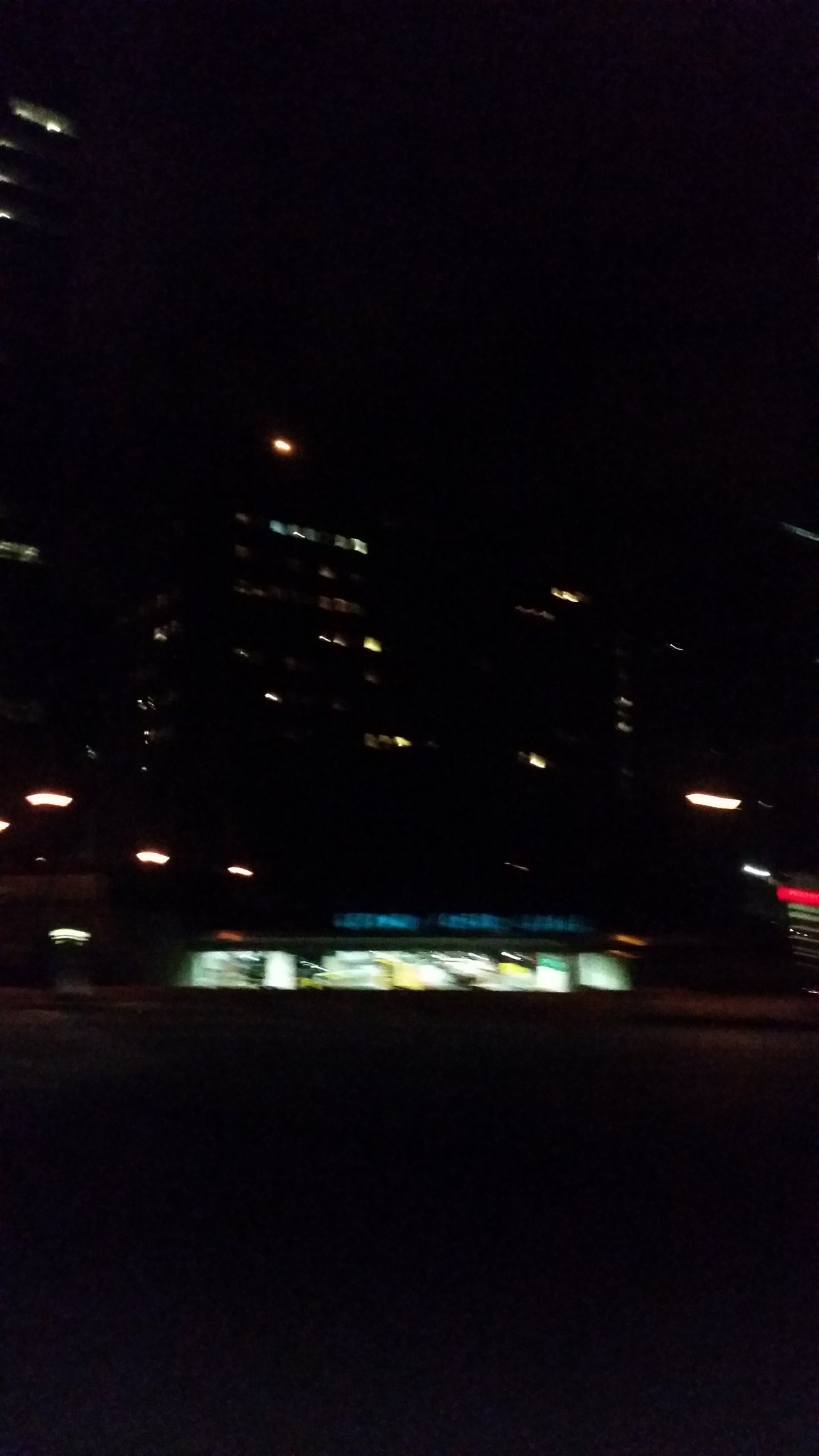In this tall, portrait-oriented photograph likely captured on a mobile phone, the night encapsulates the scene, lending an air of mystery and surrealism. The limited light conditions result in a slower shutter speed, introducing a significant amount of blur to the image. Dominating the foreground, there's a bus or perhaps an electric train car whizzing past, its swift motion further intensified by the blur. 

In the background, looming city buildings stretch upward, their presence barely discernible against the dark canvas of the nocturnal sky. The structures are only traceable thanks to the scattered illuminations pouring out from their windows. These bright squares of light, ranging from stark whites and cool blues to occasional bursts of red from streetlights, punctuate the night and provide the main sources of visibility in the photo. The upper portion of the frame is an uninterrupted expanse of night sky, emphasizing the enveloping darkness that dominates the scene.

This photograph captures the essence of urban nightlife—a blur of activity against the static backdrop of towering, nearly indistinguishable buildings, all immersed in the cloak of night.